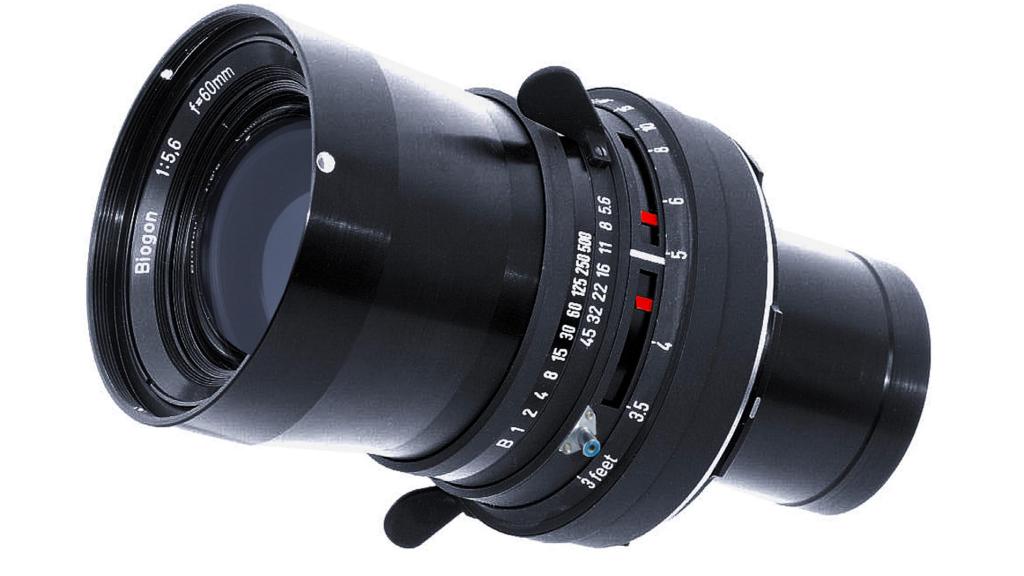The image displays a detailed, standalone black SLR camera lens on a stark white background, suitable for use in an advertisement or product showcase. This sophisticated Biogon lens features three main components: an extending lens barrel about an inch and a half long, with the brand name "Biogon" and technical details "1:5,6" and "F=60mm" prominently printed on it. Surrounding the lens are multiple control dials, including a numeric dial with the range from 1 to 500, another with settings from 45 to 56, and a gauge that likely indicates distance, marked with feet measurements ranging from 3 to 10 feet. Additionally, the control dial features a range with numbers including B, 1, 2, 4, 8, 15, 30, 60, 175, 200, 500. The lens ends with a small eyepiece extending towards the back, making the entire setup appear both functional and elegant. Numeral gradations indicate 45, 32, 22, 16, 11, 8, and 5.6, allowing for various fine-tuning options.